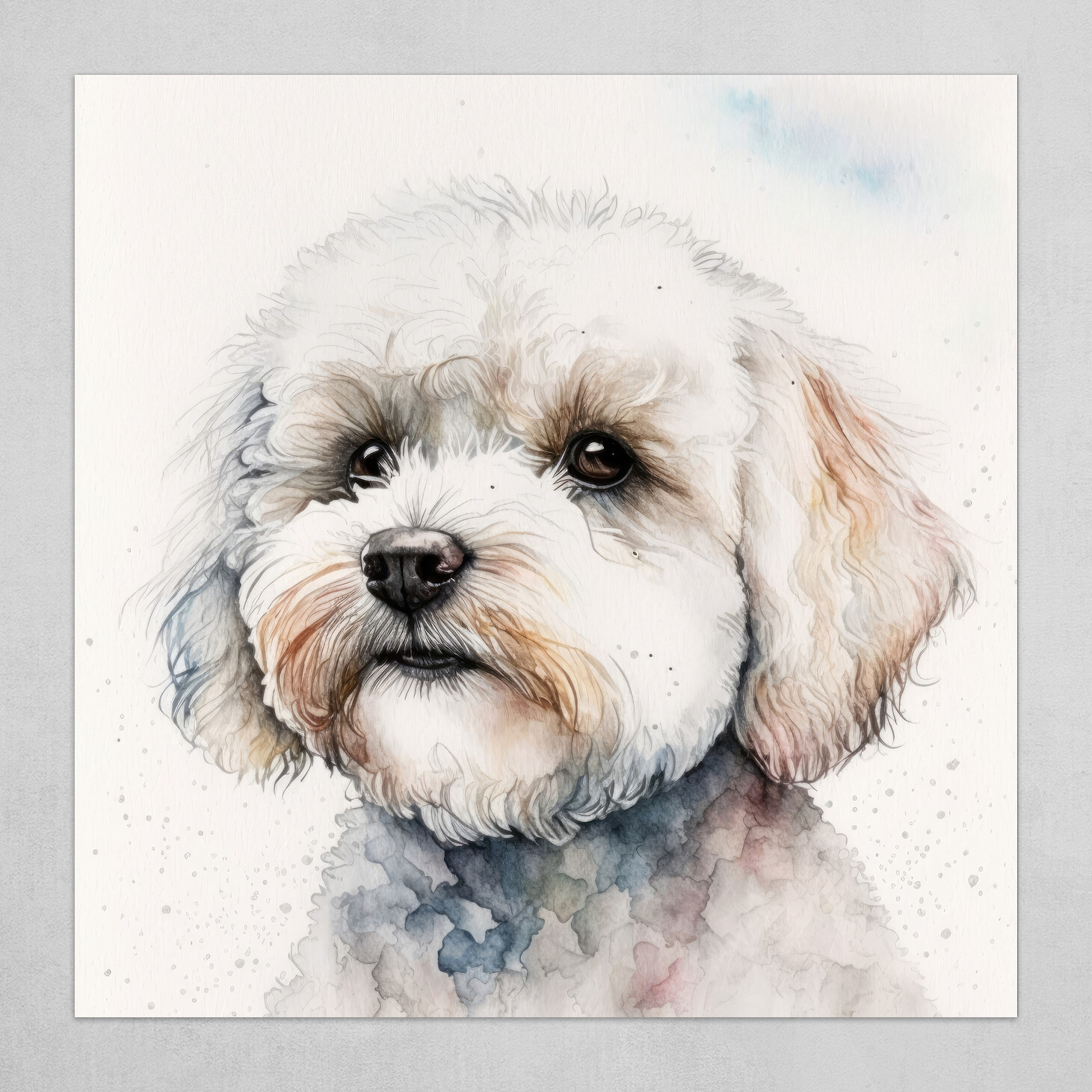This image showcases a detailed watercolor painting of a small, white dog, possibly a poodle or bichon. The dog has a well-groomed and curly coat with noticeable brownish-orange streaks around its eyes, ears, mouth, and chin, adding to its endearing appearance. Its ears hang down to its chin, highlighting the thickness and curliness of its fur, particularly around the beard area. The dog has expressive brown eyes and a black nose, giving it a cute and inquisitive look as it poses slightly to the left. The artwork features splashes of blue and pink around the ear, throat, and body, adding depth and color variation. The background of the painting is predominantly white, contrasted by a beige-colored border frame and a gray outer border. Overall, the painting vividly captures the charming essence of this small dog with its intricate use of colors and details.